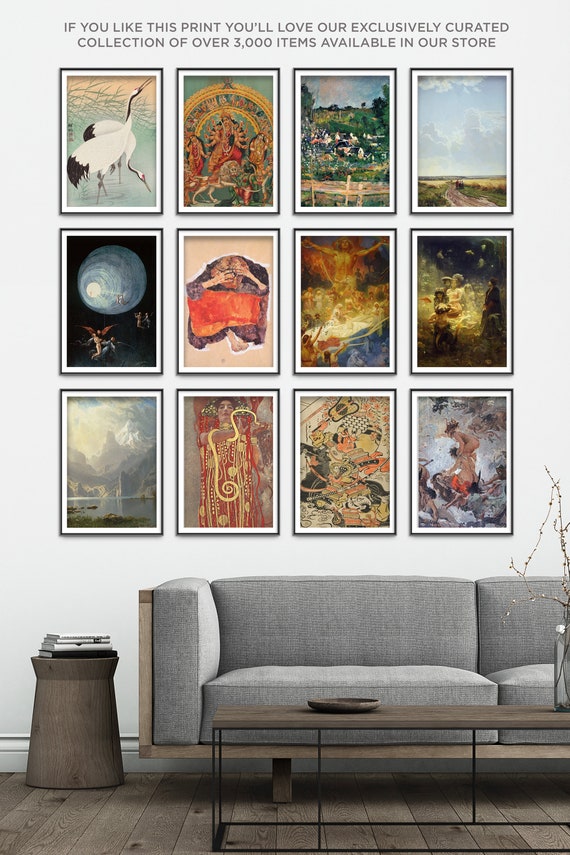This professionally taken color photograph showcases a modern, minimalist lounge area featuring a grey sofa adorned with cushions. The focal point of the room, the sofa's clean lines and simple, wood-accented design exude sophistication. Positioned in front of the sofa is a small coffee table with a wooden surface supported by thin black wrought iron, upon which rests a decorative wooden plate. To the side, a rounded side table holds a neatly stacked collection of books and a glass vase with a branch. The room boasts a darker wood floor that complements the furniture's aesthetic.

Dominating the white wall behind the sofa is a collection of 12 distinct framed pictures, each portraying unique images including landscapes, animals, and human figures. The uniform framing of these artworks ties them together visually despite their varied subjects—one features crane birds, others depict mountains, people, and abstract scenes.

Above this art display, a large, eye-catching text promotes the collection: "If you like this print, you'll love our exclusively created collection of over 3,000 items available in our store," indicating the image serves as an advertisement for a company specializing in home decor.